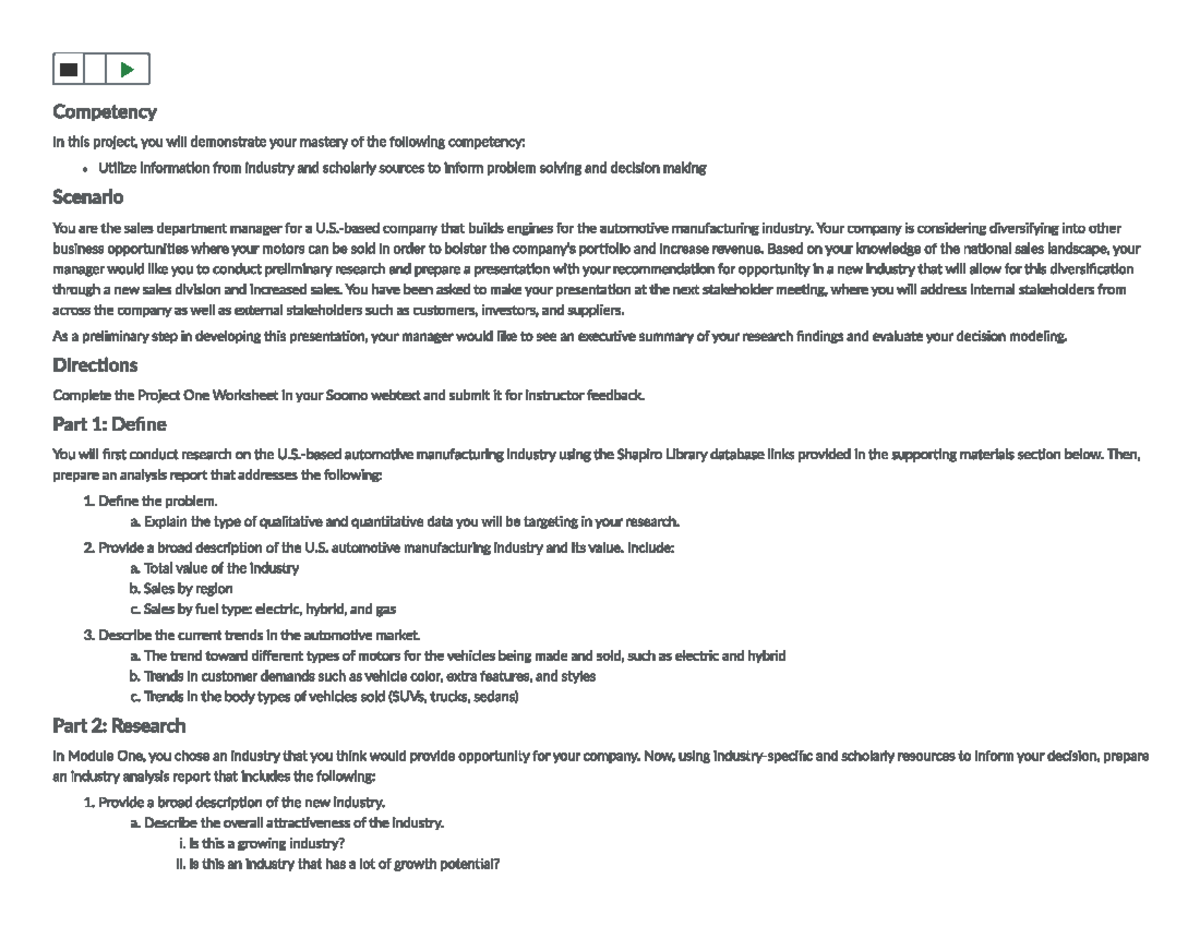**Caption:**

The image depicts a digital interface with a textual description outlining a research project centered around competency development in problem solving and decision making. The screen features three black horizontal lines and a green play button icon, followed by the term "competency." The task requires demonstrating mastery by utilizing industry and scholarly resources. 

**Project Overview:**

- **Scenario:** You are the Sales Department Manager at a U.S.-based company specializing in engine manufacturing for the automotive sector. The company is exploring diversification into new markets to strengthen its portfolio and boost revenue.
- **Objective:** Conduct preliminary research and prepare a recommendation for potential new industry opportunities, aiming for diversification.
- **Stakeholders:** External stakeholders include customers, investors, and suppliers. An executive summary of research findings is needed to assess decision models.

**Instructions:**

1. **Conduct Research:**
   - Investigate the U.S. automotive manufacturing industry using provided Shapiro Library database links.
   - Prepare an analysis report covering:
     - Problem definition.
     - Types of data (qualitative and quantitative) targeted in research.

2. **Industry Analysis:**
   - Detailed description of the U.S. automotive manufacturing industry:
     - Total industry value.
     - Sales by region and fuel type (electric, hybrid, gas).
   - Market trends:
     - Types of motors being manufactured and sold.
     - Customer preferences in vehicle color, features, and style.
     - Trends in vehicle body types (SUVs, trucks, sedans).

3. **Choosing a New Industry:**
   - Select an industry with potential for company diversification.
   - Utilize scholarly resources for an industry analysis report, including:
     - Overall industry attractiveness.
     - Growth potential and industry trends.

**Submission:**
Complete Project One Worksheet in the SOMA web text and submit it for instructor feedback. The project is part of a module aimed at defining and analyzing new industry opportunities using comprehensive research methodologies.